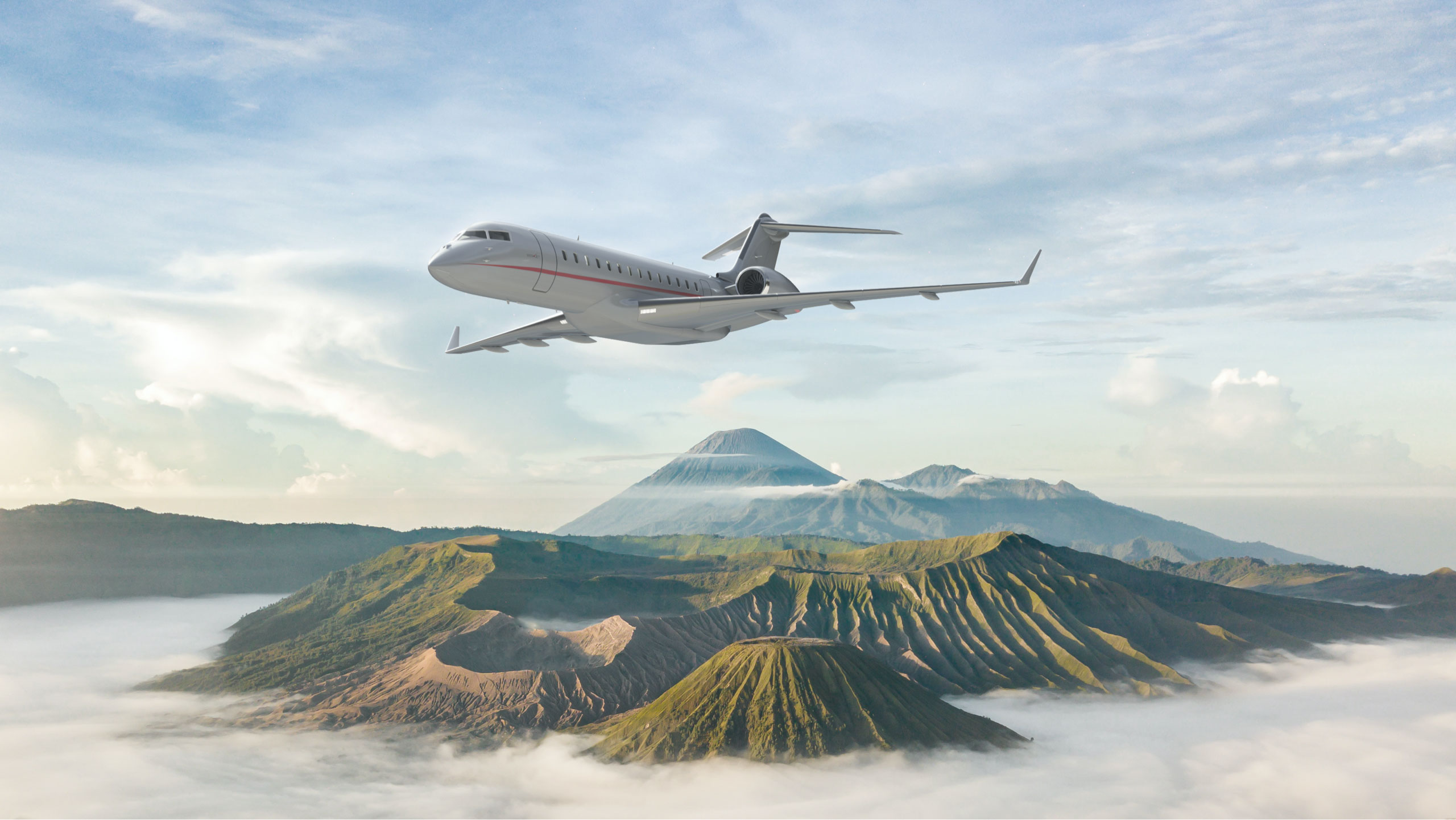This high-quality color photo captures a white passenger Learjet with a distinctive red stripe flying through a light blue sky dotted with puffy white clouds. The jet is prominently positioned in the upper center of the image, with its nose pointed towards the left. Below the plane lies a verdant island landscape, likely Hawaii, characterized by rugged, craggy terrain hinting at its volcanic origins. The island is populated with green and brown volcanoes, including a prominent cone-shaped peak in the bottom center. Thick, swirling white clouds enshroud the base of these volcanoes, creating an ethereal appearance that makes it difficult to see the land beneath. Pale light filters in from the bottom left, adding a touch of warmth to the scene.